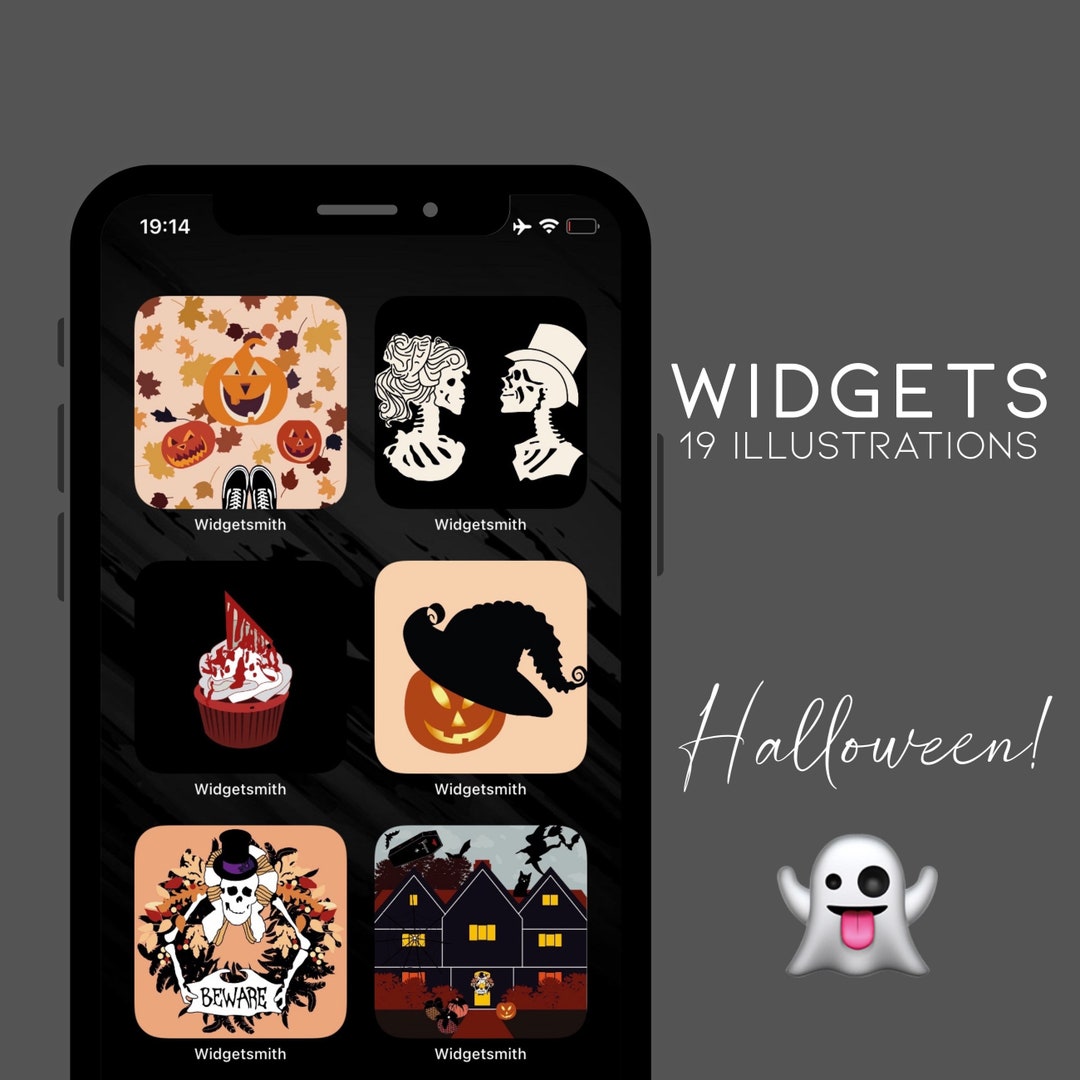This detailed and cleaned-up caption accurately describes the advertisement image for an app or widget with a Halloween theme:

"Advertisement for a Halloween-themed app/widget. The image features a phone on a gray, slashed-line background. The phone displays various app icons, all labeled 'Widget Smith', showcasing different Halloween-themed illustrations. These include pumpkins, a pair of Converse sneakers with autumn leaves, two skeletons with fancy wigs and hats facing each other, a pumpkin with a witch's hat, and a sign saying 'Beware' made from bones held by a skull. There's also a scene with trick-or-treaters approaching a house. Next to this, the text reads 'Widgets, 19 illustrations' followed by 'Halloween' with a ghost emoji sticking its tongue out. To the left of the pumpkin with a witch's hat, there's a red velvet cupcake with white frosting and a red flag, the text on which is difficult to read. The phone screen shows the time as 19:14 at the top left corner. Overall, the gray background complements the Halloween aesthetics of the displayed widgets."